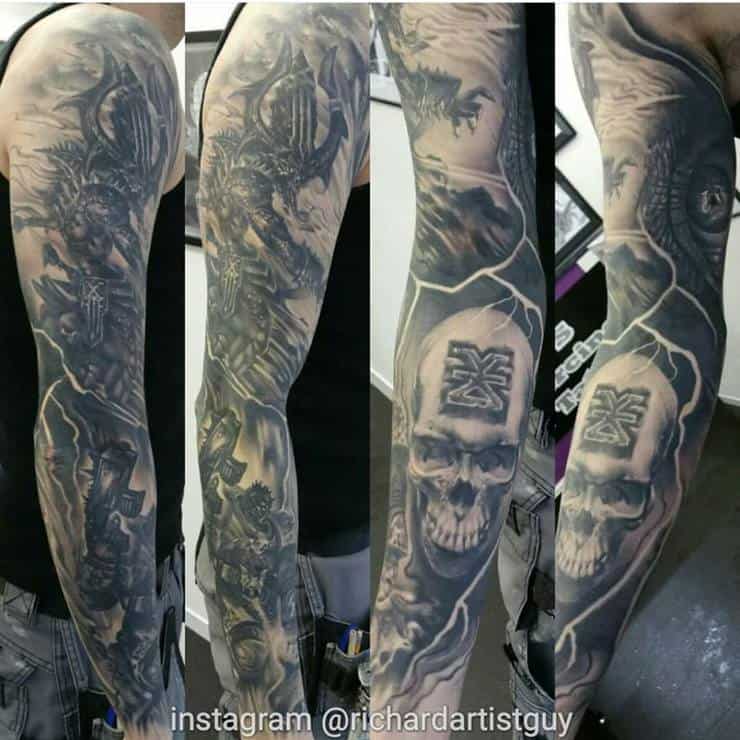The image is a detailed collage consisting of four rectangular frames, each depicting a tattooed arm of a man wearing a black sleeveless vest. The collage shows both arms fully covered in intricate black and grey tattoos, captured from four different angles. One arm features a depiction of a demon creature, a detailed skull with an X on its forehead, and significant shading and dark shadows. The other arm appears to illustrate a chaotic battle scene, including a soldier holding a gun and what resembles dragons or comic book characters. The background of the images is a white wall adorned with photo frames. At the bottom of the collage is a watermark that reads "Instagram @RichardArtistGuy."